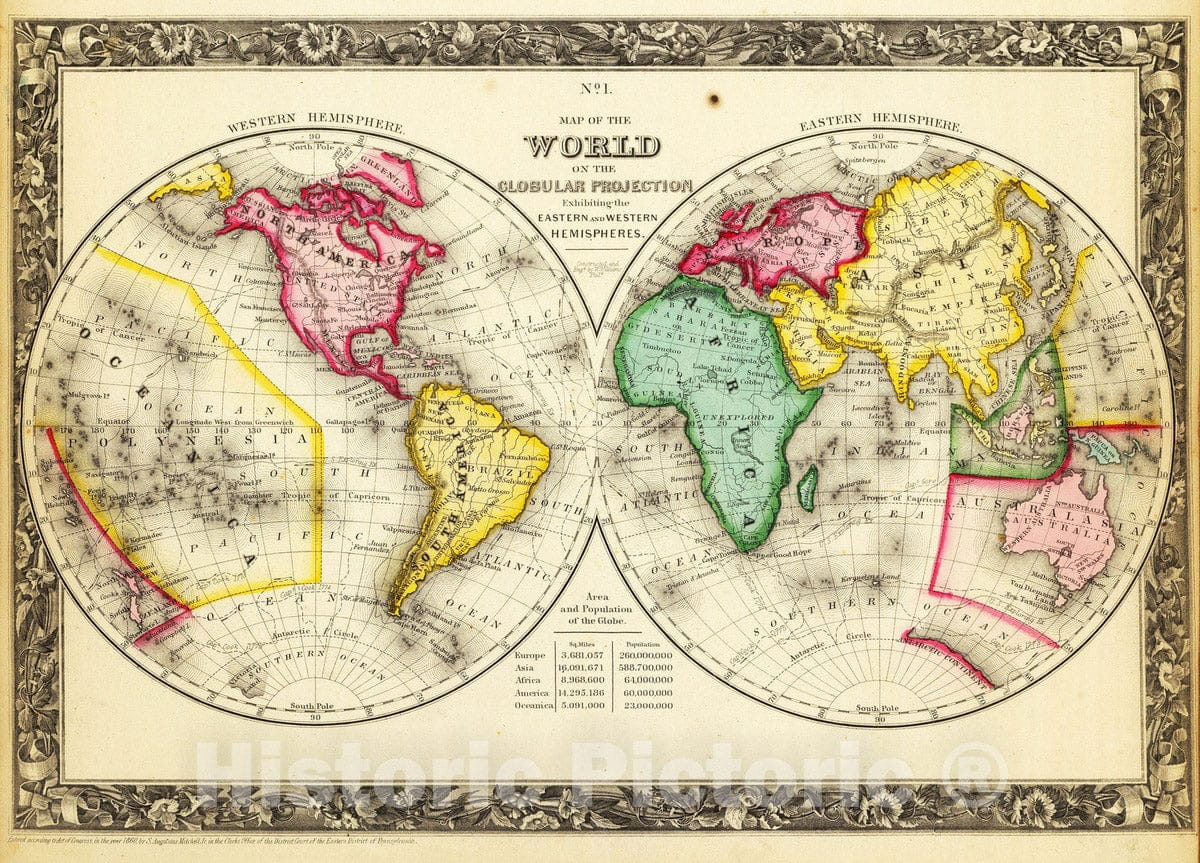This image depicts a meticulously enhanced, multi-colored vintage map of the world, presented in a horizontally rectangular format. Centered on the map are two adjacent globes—one labeled "Western Hemisphere" on the left and the other "Eastern Hemisphere" on the right—accompanied by the title "Map of the World on the Globular Projector" with the subtitle "Establishing the Eastern and Western Hemispheres." The map is bordered by three distinct frames: a clear outer border, a very ornate middle border, and a thin inner border. The background is a light brown off-white hue. There’s a watermark at the bottom stating "Historic Pictoric Registered Trademark."

The Western Hemisphere globe features landmarks like North America in red, South America in yellow, and includes Alaska, Nova Scotia, Canada, the United States, the Caribbean, and stretches of the Pacific Ocean marked in yellow stripes. The Eastern Hemisphere globe showcases Africa in green, Asia and Eurasia in yellow, Europe in red, and Australia in pink, positioned at the far right bottom. Additionally, Antarctica is depicted in pink and populated regions and oceanic areas are distinctly highlighted with various vibrant colors, making the old map visually striking and informative.